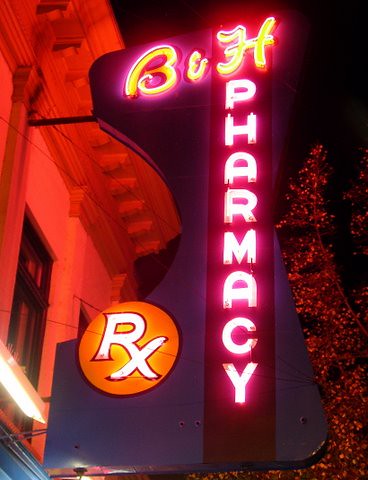A night-time photograph beautifully captures a vintage building adorned with intricate architectural details. The image, taken from a low angle beneath a dark sky, showcases a glowing neon sign affixed to the facade. In vibrant yellow script, the letters "B and H" are prominently displayed. Running vertically in crisp white neon, the word "Pharmacy" draws the eye downward. Adding a nostalgic touch, an orange circle illuminated with neon light encapsulates the white "RX" symbol, further highlighting the building's historical charm. The juxtaposition of the neon glow against the night sky creates a mesmerizing and timeless scene.